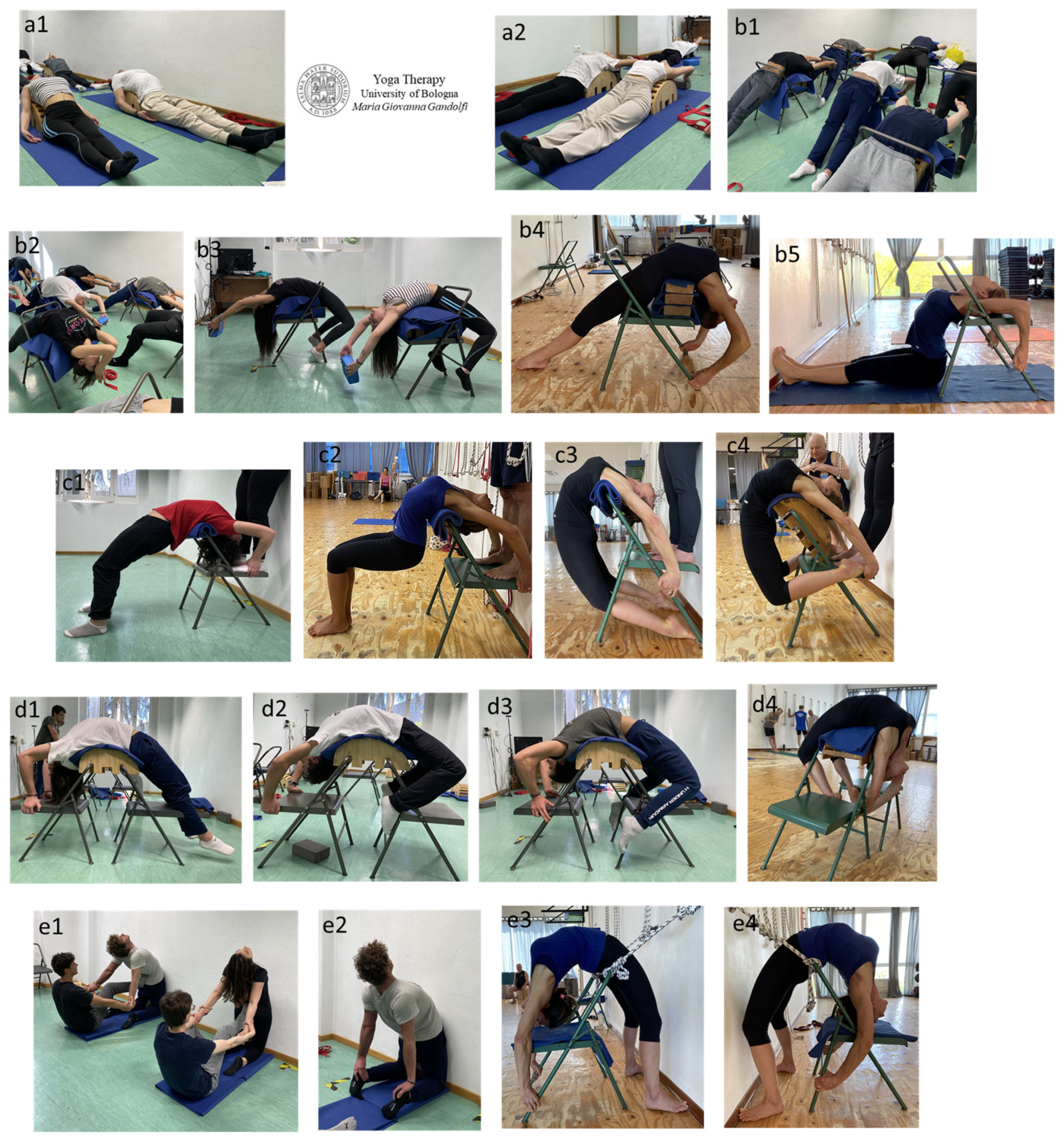In this image, a group of individuals is seen engaging in various yoga therapy exercises, overseen by the University of Bologna, specifically designed by Maria Giovanna Ganzolfi. The participants are positioned both on blue mats and using green folding chairs to aid in their stretches, indicating a therapy session possibly aimed at back strengthening and relaxation. The setting appears to be an instructional or therapeutic environment, likely a classroom, as evidenced by the detailed display of multiple sequential photos labeled from A1 to E4. These photos illustrate a variety of yoga poses, many of which involve backward bending and the use of ropes, chairs, and walls—all tailored to help individuals with potential back issues. The crest from the university, along with the title Alma Mater Studiorum and an indistinguishable date, is prominently featured, adding an official touch to the therapeutic practice being showcased.